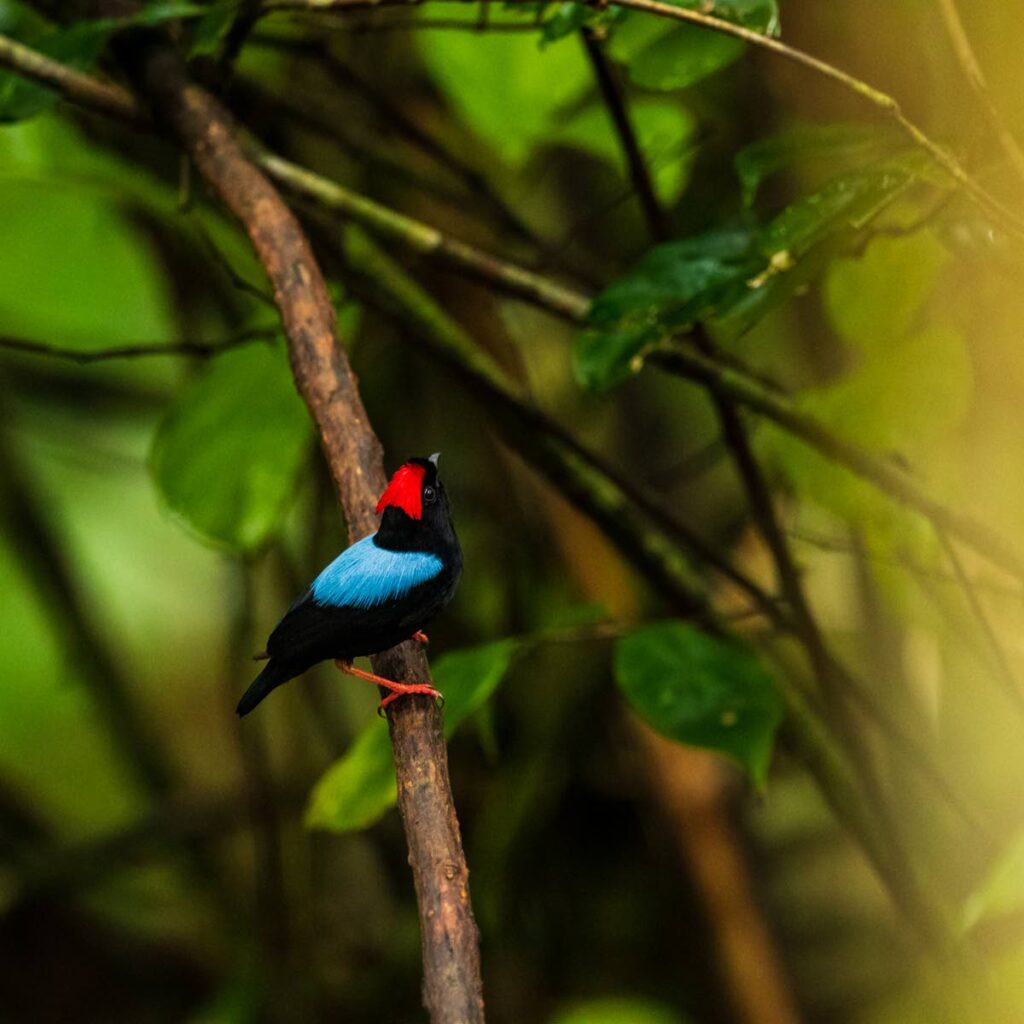The image is a large square close-up of a small bird perched on a thicker brown tree branch that extends from the upper left corner down towards the middle of the picture. The bird has predominantly black feathers, with a vivid blue coloring on its back and wings, and a bright orange-red patch on its head. Its beaded right eye and short beak are visible as it gazes upwards and to the right. The bird's orange feet grip the branch. The background is a blurred mix of green leaves and thin branches, with a noticeable yellowish light on the right side, likely due to sunlight filtering through the foliage. The left side of the background is predominantly green with more green leaves.